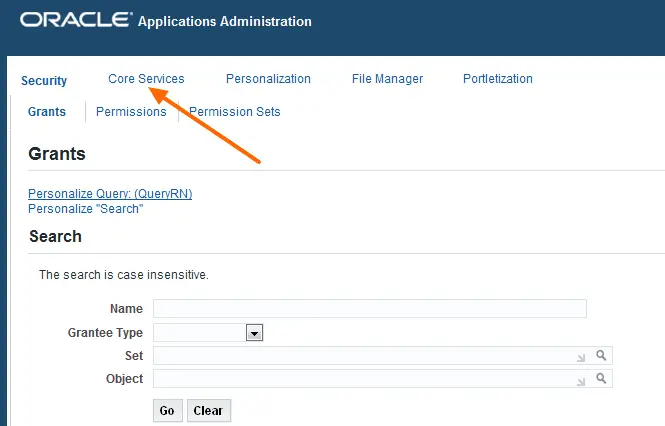This image prominently features a user interface for an application, likely related to web design or application programming. Presented in landscape orientation, the image lacks clearly defined external borders and showcases a mix of blue and white tones.

At the top, there's a long, rectangular blue header with the word "Oracle" displayed in white font on the left side, accompanied by a trademark symbol. Adjacent to it are the words "Applications Administration." The header is delineated by a thin border running down its left side, and beneath it lies a large white box.

On the top left of the white box, two rows of tabs are visible. The first row contains tabs labeled "Security" (highlighted in a darker blue), "Core Services," "Personalization," "File Manager," and "Portalization." The second row includes "Grants," "Permissions," and "Permission Sets," with an orange arrow pointing upwards towards the "Core Services" tab.

Below these tabs, there is a section marked "Grants," identified by a thin green line, and contains two clickable links: "Personalized Query" and "Personalized Search." Below this, another header labeled "Search" emphasizes that the search functionality is case-sensitive.

At the bottom of the white box, there is a form section with fields labeled "Name," "Grantee Type," "Set," and "Object," accompanied by "Go" and "Clear" buttons for executing or resetting the search, respectively.

Overall, this detailed user interface appears to be designed for managing various administrative aspects, with a focus on permissions and personalized queries and searches.